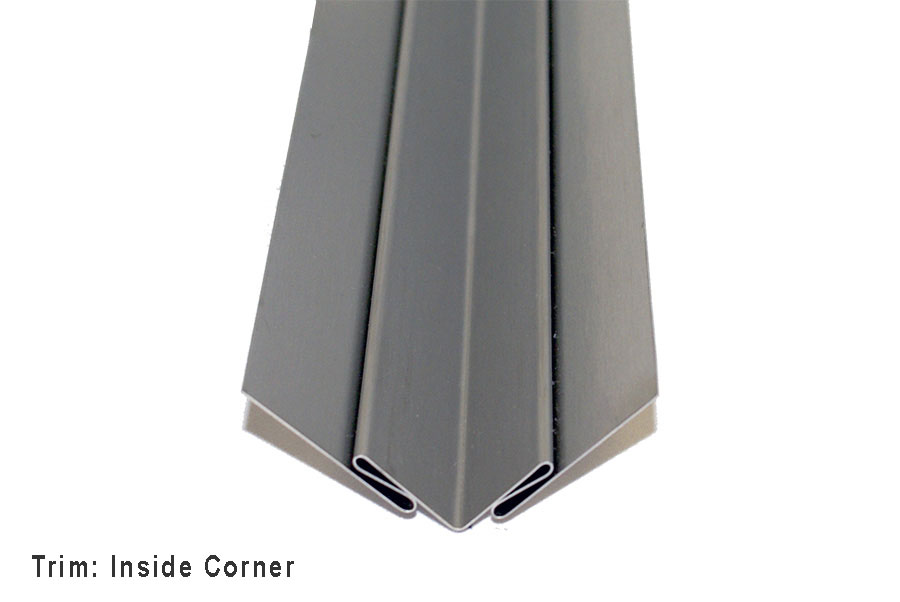The image features a large, arrow-shaped piece of metal trim positioned centrally and pointing downward against a completely white, empty background. The dark silver trim has multiple folds, creating four distinct sections with subtle shadows along its edges. The image appears to be taken in a minimalist setting, possibly for an advertisement from a home improvement store or a website like Lowe's or HomeDepot.com. In the bottom left corner, there's text that reads "trim inside corner." The composition highlights the metallic object prominently while maintaining a clean and simple backdrop.